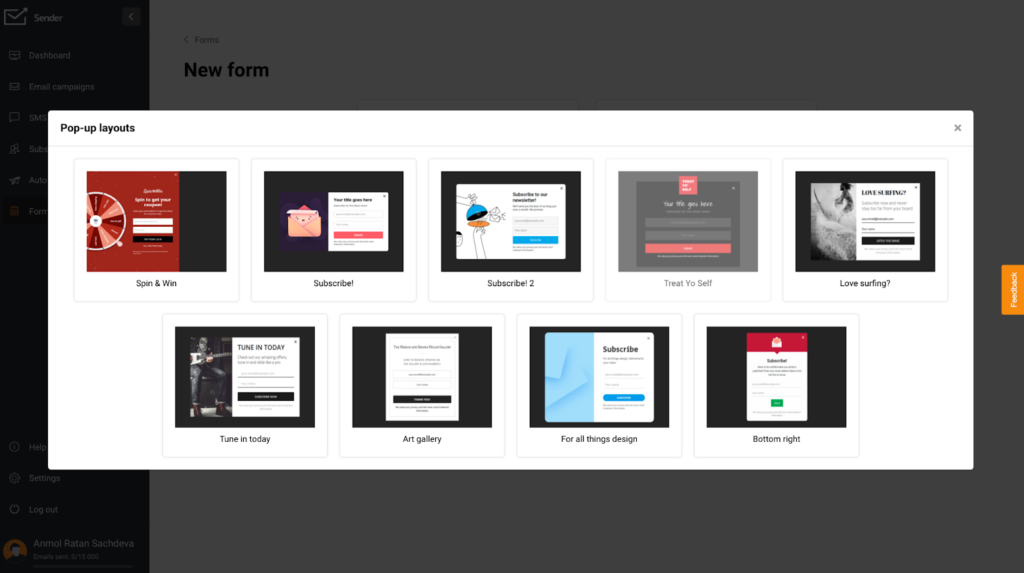In this image, a user interface displays various pop-up layouts. The scene is primarily divided into two distinct rows, each containing several squared boxes with accompanying images and text descriptions.

In the top left corner of the image, the title "Pop-up Layouts" is written in black text. Directly below this header, the first row contains five different boxes, each labeled with unique descriptions:

1. The first box on the far left is labeled "Spin and Win" and features an image of a lottery wheel.
2. Next to it, the second box displays "Subscribe" above an image of a sign-up area featuring a bear.
3. The third box is also labeled "Subscribe" but has a sign-up image depicting what appears to be a hamburger.
4. The fourth box says "Treat Yourself" and contains a sign-up image with the text "Love Surfing."
5. The fifth and final box in the top row says "Tune In Today" and showcases an image of a man holding a guitar.

The second row features another series of boxes with descriptive labels:

1. The first box says "Art Gallery," which includes a sign-up page.
2. To the right of it, the box reads "For All Things Design," indicating another subscribe page.
3. The last box on the bottom row, labeled "Bottom Right," displays a sign-up page.

In the bottom right corner of the image, there is a small orange box on its side, labeled "Feedback."

The background of the user interface is mainly white, providing a clean and minimalist look. However, the left side of the image contrasts with a darker black background.